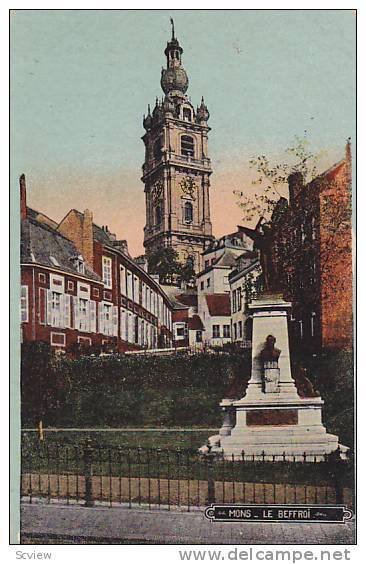This color illustration, likely depicting a scene in a European city, seems to be set in France, as suggested by a partially legible street sign reading "Mont Libre." The portrait-format image showcases a diverse urban landscape with a focus on a grand central structure. This tall, narrow stone building, topped with a dome-like spire and possibly housing a clock, commands the background. Atop this building is a large statue featuring an angel with wings.

In the midground, two rows of apartments are visible. The left side comprises two-story, red-brick buildings with numerous white windows and shutters, a gray peaked roof adding to their charm. On the right side stands another red-brick building, contributing to the city's densely built environment.

In the foreground, a brass-like statue mounted on a white base is enclosed by an iron gate in a park-like setting, surrounded by grass. Low metal fences also delineate sections of this area. The overall scene exudes a somewhat dark and muddy palette, enhancing the aura of an old-world European cityscape, with chimneys and windows punctuating the distant buildings. The bottom of the image appears to reference a website, "www.delcampe.net," indicating its possible origins from an online source.